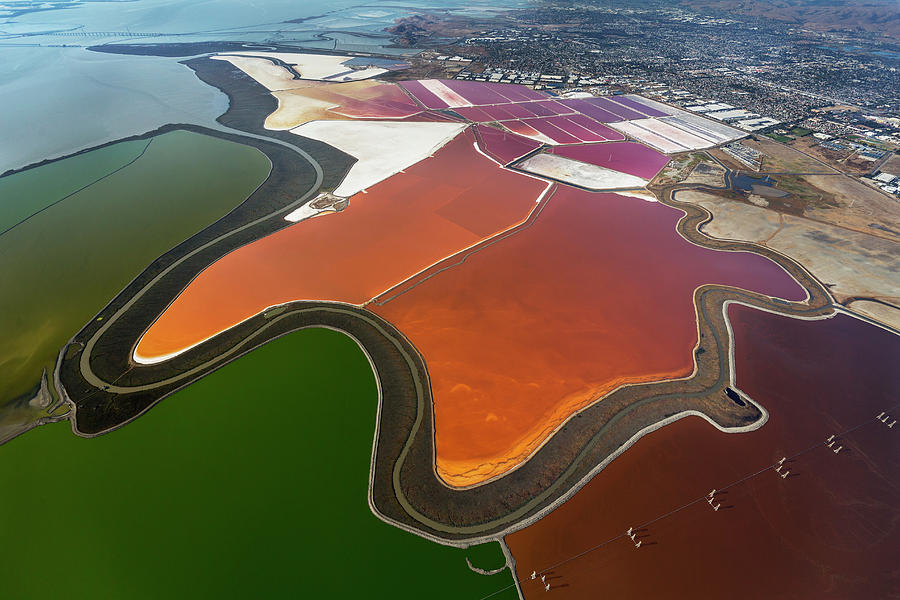This aerial photograph captures a strikingly colorful landscape that blends natural and urban elements. Dominating the center of the image is a vibrant patchwork of red, orange, and yellow hues, bordered by stark white sections and encircled by a dark pathway that resembles a road. The left side of the image features a solid green area that intriguingly contrasts with the more recognizable blue water visible at the top of the frame. The top right portion reveals a cluster of tiny buildings, suggesting the presence of a town or city. The entire scene is characterized by a variety of shapes, including squiggles, blocks, rectangles, and triangles, amidst sections of dark brown-orange bordered in white. The overall effect is both beautiful and puzzling, presenting a mosaic-like landscape that blurs the lines between land and water, nature and urbanization, and leaves the viewer in awe of its vibrant yet enigmatic character.